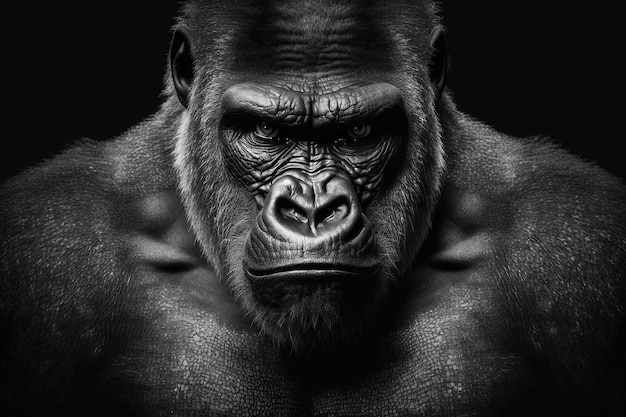This highly detailed digital illustration, almost photographic in its realism, captures the intense visage of a gorilla staring directly at the viewer. The gorilla's face, front and center in the composition, is rendered with intricate detail, featuring furrowed brows, textured skin, and partially shadowed eyes that convey a serious, intimidating expression. The black background enhances the striking black-and-gray tones of the gorilla’s fur, which is particularly noticeable around the chin and ears where some gray or white hairs are visible. The gorilla’s closed mouth has a subtle curve, adding to its formidable presence. The image includes the shoulders and part of the torso, highlighting muscular details around the shoulder and pectoral areas, as well as some scale-like skin textures under the chin. Overall, the close-up perspective, combined with the gorilla’s intense stare, creates a powerful and commanding image.